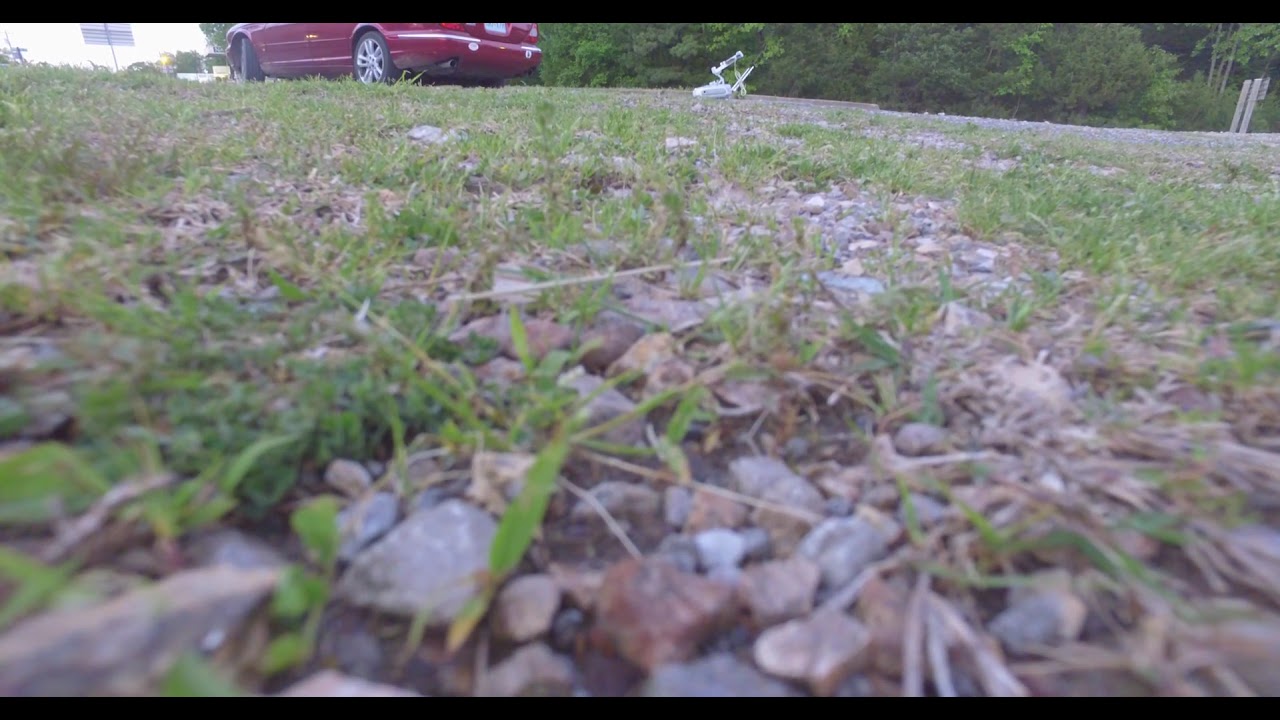The photograph, taken from ground level, captures a detailed scene featuring an up-close view of rocks and grass, with some trash and dead grass interspersed. The extreme foreground is somewhat blurry due to the close proximity, yet outlines of these elements remain discernible. Moving towards the midground, a red car, the back half of which faces the viewer, is parked slightly to the left. This car is a regular, burgundy-red vehicle, partially revealing its two rear wheels, trunk, and part of the license plate. Adjacent to the car, on the right, appears to be white debris, possibly a discarded object like a lawn chair. Centered behind the car stands an indistinguishable piece of machinery or possibly a drone. The backdrop of the image, stretching across the top, is composed of the faint outlines and tops of trees and bushes, suggesting an outdoor setting. Additionally, towards the far right, a sign is visible, showing only its back and the supporting posts. The scene, captured in a horizontal rectangle format, brims with natural hues of gray, brown, green, along with the prominent red of the vehicle, all under the daylight, potentially late in the afternoon.